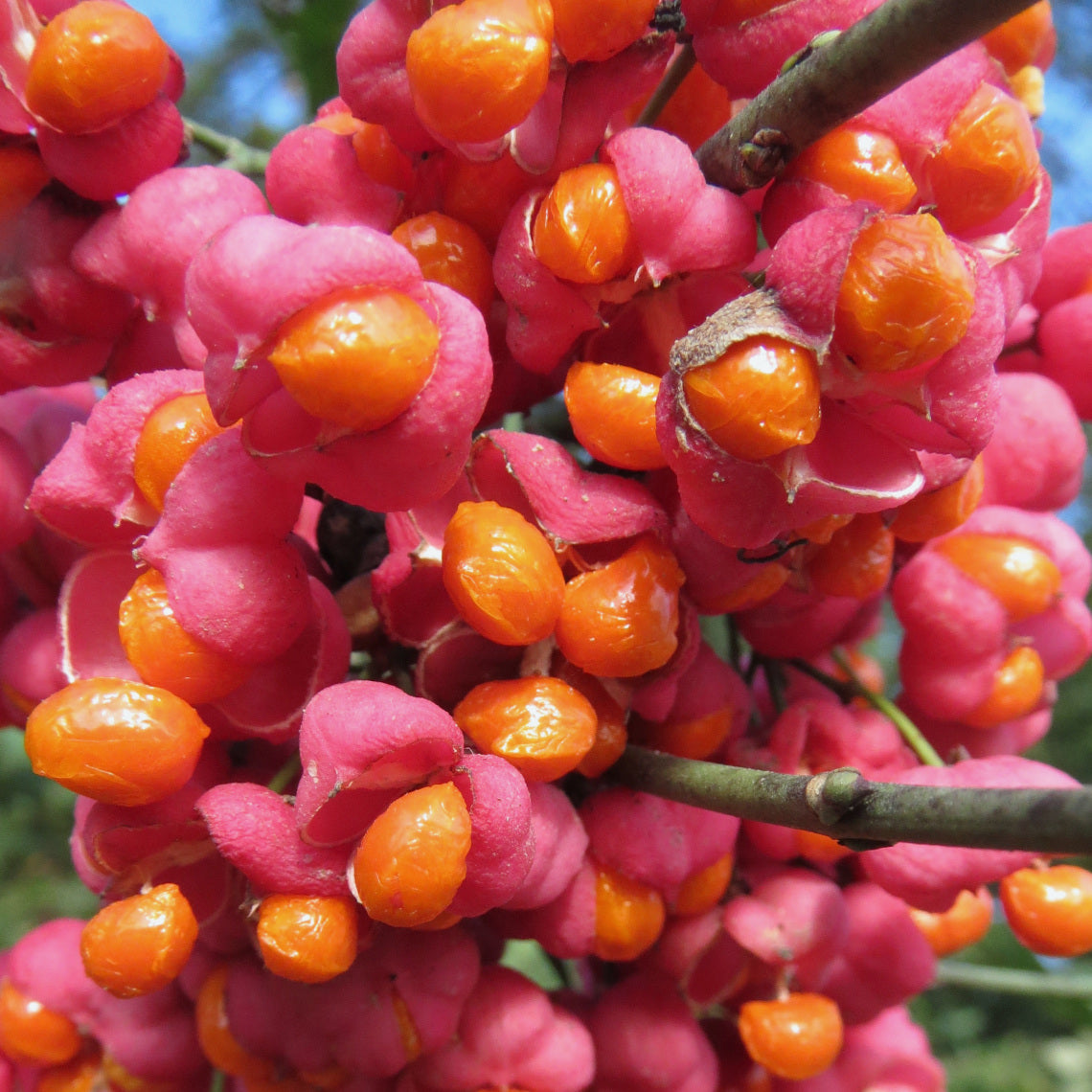The image centers on a cluster of vibrant pink flowers in full bloom, drawing the viewer's attention. The flowers are adorned with glossy, orange seed pods or fruit, reminiscent of miniature oranges, emerging from within their petals. The main focus is sharply on these flowers, while slender branches extend from the right, supporting the floral display. In the background, a beautifully blurred scene of ground vegetation and tree silhouettes merge softly into the backdrop, with patches of blue sky peeking through the foliage, adding a serene ambiance to the composition.